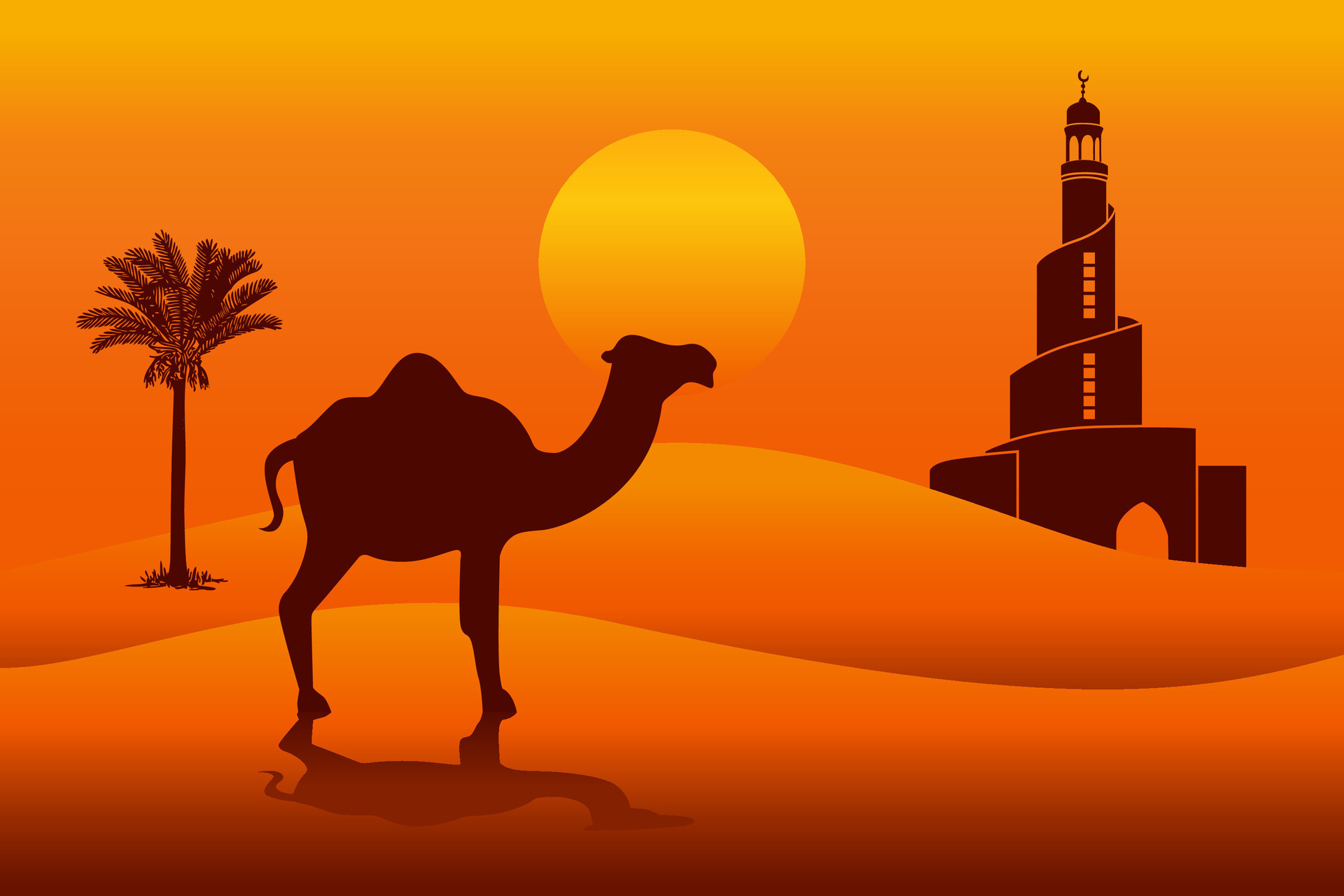This image is a simple yet captivating vector illustration, featuring the striking silhouettes of various elements set against the backdrop of a desert sunset. Dominating the center is a sturdy brown camel with a single, prominent hump. The camel's head, level with the hump, faces right, and it casts a subtle shadow on the rolling dunes beneath it. These dunes, depicted in shades of light gold-orange that transition to bright orange and eventually dark brown, suggest a sunlit, sandy landscape. To the left stands a palm tree with foliage concentrated at the top and some brush near its trunk. Further enriching the scene, to the right is an architectural silhouette resembling an Asian temple with a spiral design that ends in a crescent moon-like spire. Above the camel, a perfectly round sun in the background glows a soft yellow, fading into darker shades towards its top and bottom. The sky, vibrant in hues of yellow at the top gradually blending into orange, frames the entire scene, evoking the warm ambiance of a desert at sunset.